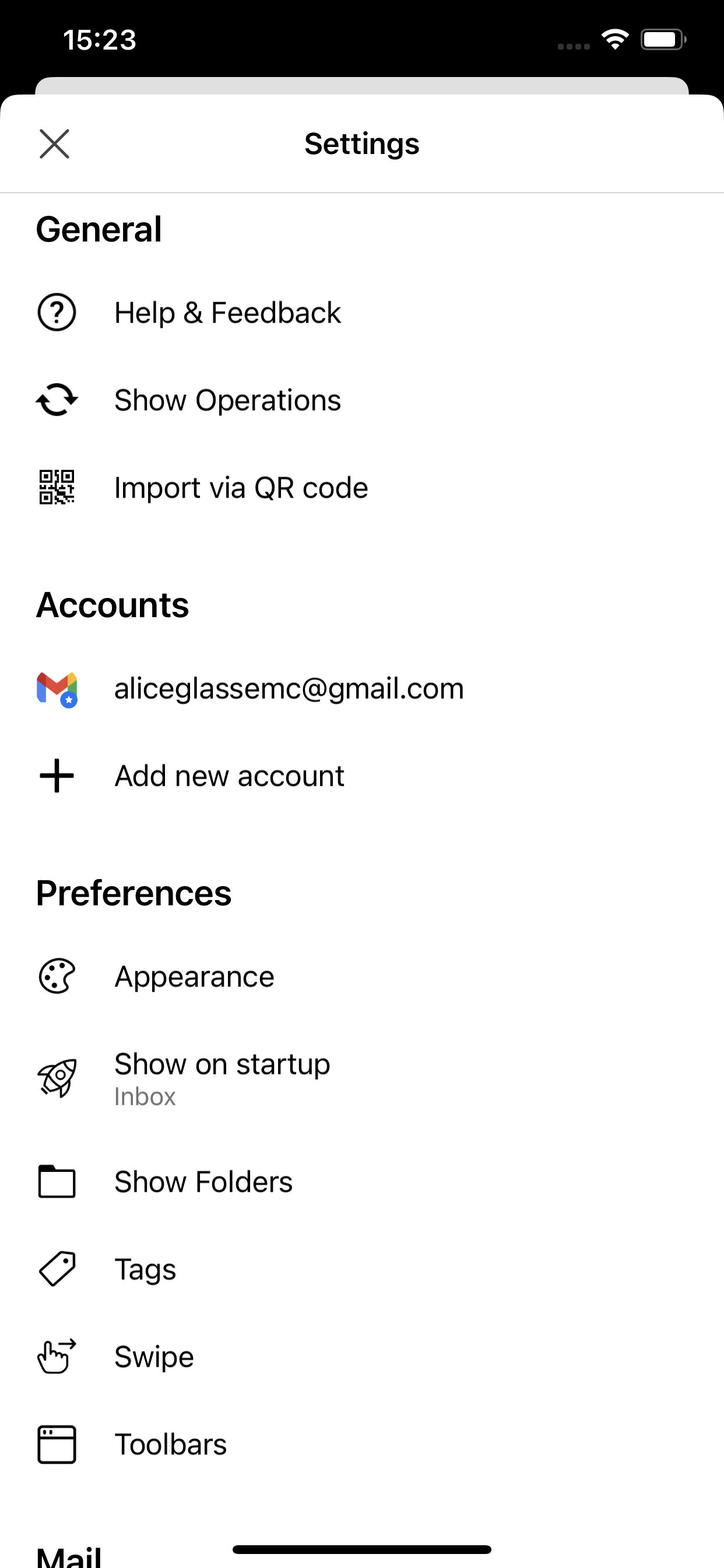The image is a screenshot from a cell phone depicting the settings screen. At the top, there's a black rectangle featuring the time, "15:23," displayed in white text on the left side and the battery indicator along with the Wi-Fi icon on the right side. Beneath this black bar, the majority of the screen is a large white rectangle.

In the upper left corner of the white section, there's a small gray "X," with the word "Settings" next to it in bolded black font. Directly below, the section is titled "General" in bold black text. This category has three items listed: "Help and Feedback," "Show Operations," and "Import via QR Code," each accompanied by a small icon to their left.

Further down, another section is labeled "Accounts" in bold black text. This part shows an email address, aliceglassemc@gmail.com, with an associated icon on the left, followed by the option to "Add a New Account," also with an icon.

Below the accounts section is a "Preferences" category, distinctly labeled in bold black text. The preferences list includes "Appearance," "Show on Startup," "Show Folders," "Tags," "Swipe," and "Toolbars," each item accompanied by a corresponding icon to the left.

Near the bottom of the screen, partially visible, is part of another section labeled "Mail" in bold black text. To the right of the "Mail" label is a thick horizontal black line, which is partially cut off at the bottom edge of the screenshot.